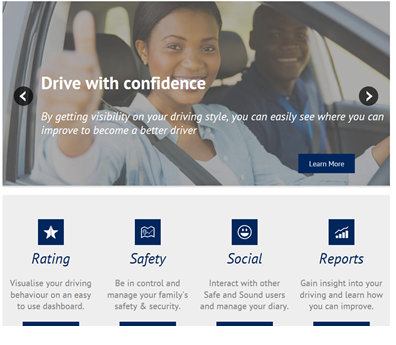This promotional image for a website showcases several features to enhance driving confidence and safety. The main background image at the top features a young woman with darker skin, black hair, and a blue shirt, driving a car and giving a thumbs up out the window. She is wearing a seatbelt, and beside her, a young man in a navy blue shirt is smiling. Overlaying this image in white text is the slogan: "Drive with confidence. By getting visibility on your driving style, you can easily see where you can improve and become a better driver." A blue "Learn More" button is located in the bottom corner.

Beneath the main image are four categories, each highlighted with blue icons and descriptions: 
1. **Rating** - Represented by a star icon, this feature allows users to visualize their driving behavior on a user-friendly dashboard.
2. **Safety** - Symbolized by a map icon, this category emphasizes the ability to manage the safety and security of your family.
3. **Social** - Denoted by a smiley face emoji, it encourages interaction with other users and the management of a driving diary.
4. **Reports** - Indicated by a graph icon, this section provides insights into your driving habits and tips on how to improve.